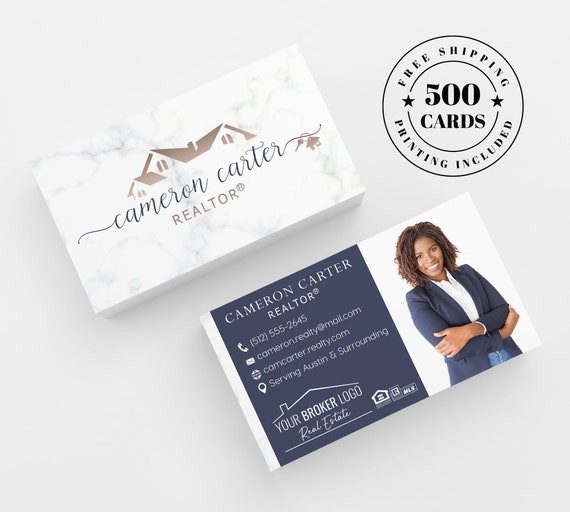This advertisement showcases a set of business cards for Cameron Carter, a realtor. The photographic image displays both the front and back designs of the cards against a clean, white square background. A prominently positioned circular graphic in the upper right announces "500 cards, printing included, free shipping," bordered with stars.

The first business card features a marbled background with a stylized rooftop logo. Cameron Carter's name appears in elegant cursive, adorned with a keychain featuring a house-shaped ornament, symbolizing her profession. Beneath her name, the title "Realtor" is inscribed in tan, with a registered trademark symbol.

The second card presents a professional portrait of Cameron Carter, an African-American woman in a blue blazer, jeans, and a white collared shirt, smiling confidently with her arms crossed. Adjacent to her photo, a dark blue text box with white font details her contact information: Cameron Carter - Realtor, phone number, email address, website, and a note indicating that she serves Austin and the surrounding area. The "Your Broker Logo" and a key-shaped logo are also included.

This detailed design highlights Cameron Carter's professional branding while emphasizing the quality and value of the advertised business card printing service.